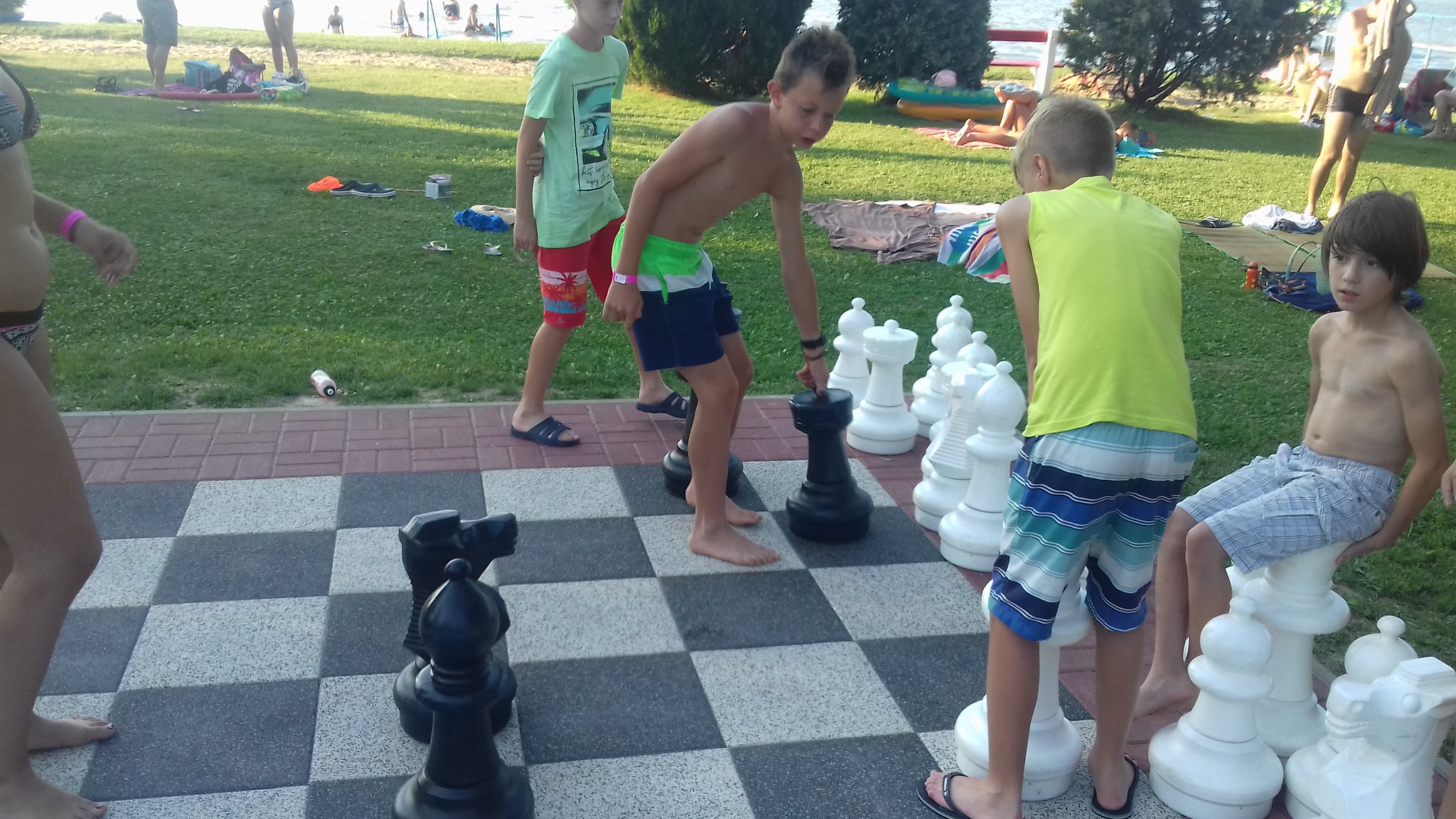In a large, green park filled with manicured grass, small trees, and scattered shrubs, several groups enjoy picnics, drinks, and sunbathing. The center of attention in this lively setting is a sizable outdoor black and white chessboard, measuring roughly 20 feet by 20 feet, entrenched in a brick-bordered concrete pad. The chess pieces, made of sturdy plastic and reaching about two feet tall for the pawns, scatter across the board rather haphazardly, indicating play rather than a structured game. Among these, four children approximately ten years of age are engrossed in imaginative play. One child is perched atop a queen piece, another is interacting with a bishop, while a third is seen tugging a black pawn. Meanwhile, an adult woman, dressed in a bathing suit, observes the scene, adding to the atmosphere of casual enjoyment and recreation in the expansive park.